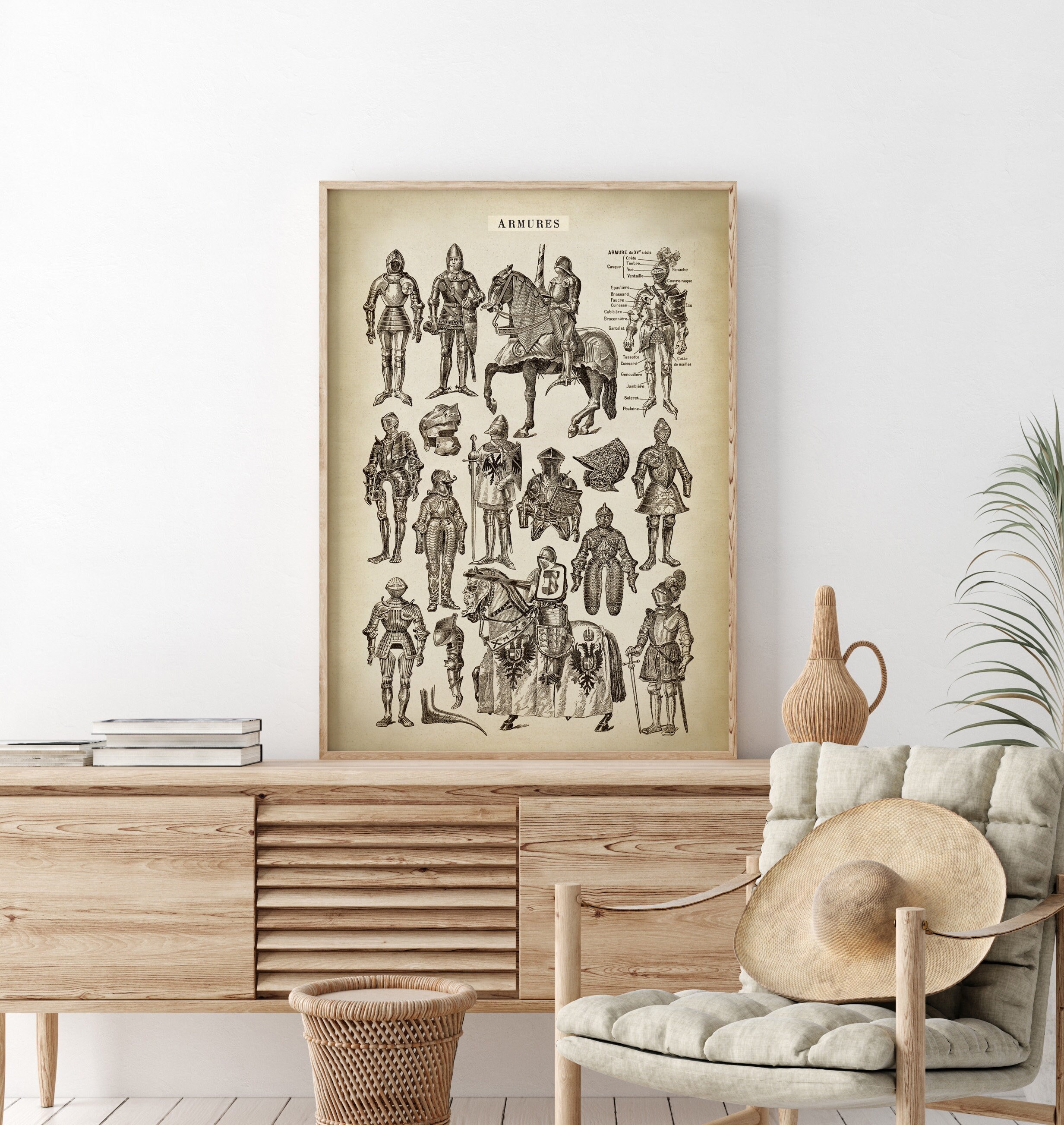The indoor scene depicts a serene room with white to grayish-white painted walls. At the center of the setting is a wooden table, on which rests an aged, framed illustration featuring knights on horseback in military attire, evoking an older era. The yellowed paper of the framed image is darkened at the corners, adding to its vintage feel. Leaning against the wall, the picture awaits hanging.

Adjacent to the table stands a wooden-framed chair with a beige, tufted cushion, adorned with a hat. Beside it, there is a wicker waste paper basket, often mistaken for an ottoman, adding a rustic touch. To the right is a light wood cabinet holding a small collection of books, with a planter visible on the right-hand side adding a touch of greenery to the room. A container with a handle is also situated on the cabinet, contributing to the room's functional yet cozy ambiance.